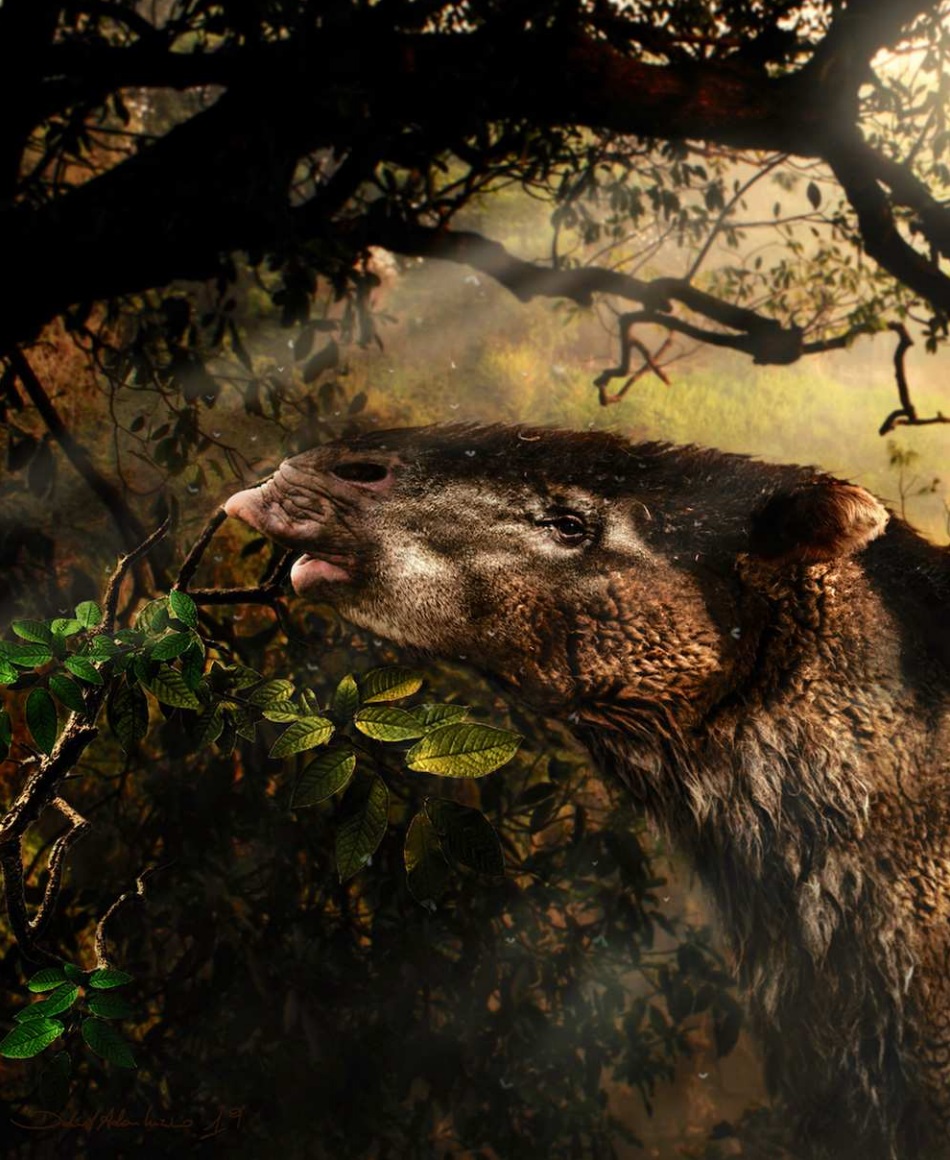The image depicts a fantastical woodland scene, resembling an artistic painting or digital rendering rather than a true photograph. Central to the composition is an enigmatic, llama-like creature with an unusual blend of light and dark brown fur, topped with a thick black mane that drapes over part of its face. The animal’s head and neck are prominently featured, with one eye, a portion of its snout, and its nostrils clearly visible. The creature appears to be reaching up towards a tree branch, possibly to eat the vibrant leaves of varying green shades, which cascade from the branch that stretches overhead. The setting is a dense forest with an array of brown branches and green foliage, shrouded in a hazy, dark ambiance. Sunlight pierces through the canopy in fragmented beams, illuminating parts of the scene and casting intricate shadows on the animal and its surroundings. The blurred background, filled with indistinct trees and foliage, enhances the mystical and otherworldly quality of the image, suggesting it depicts a creature that may not exist in reality.